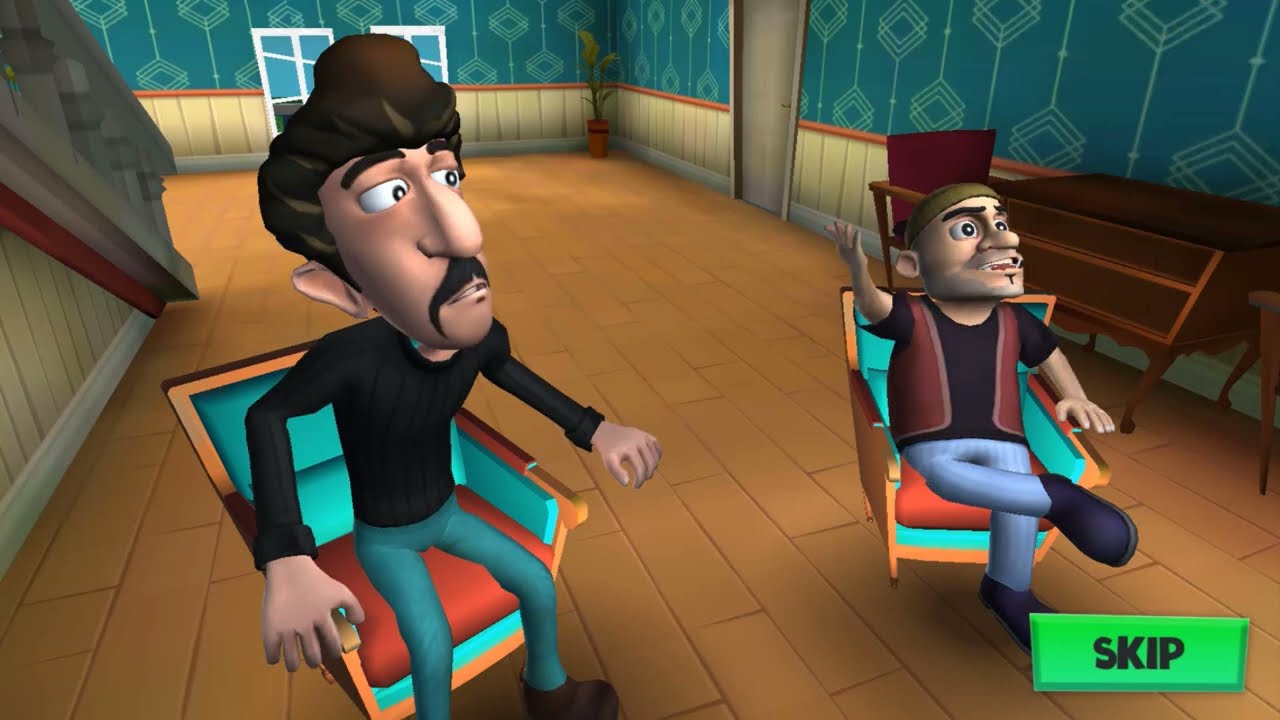The image depicts a computer-rendered, animated scenario featuring two men seated in ornate chairs within a room. Both men are facing the viewer. The man on the left is slightly rotated towards the right, dressed in a black long-sleeve shirt, blue jeans, and brown shoes. He has a prominent black mustache and brown voluminous hair. The man on the right, wearing a black t-shirt under a red vest, has lighter blue jeans and black shoes. He dons a brown beanie, sports a small goatee, and has his right arm raised as if questioning, with his left hand resting on the armrest. His right leg is casually crossed over his left. Both chairs feature blue fabric with red cushions and wooden accents.

The background showcases blue walls adorned with a white design that includes a line with staggered stars. Below this, light brown wooden paneling with white trim accents the lower portion of the wall. A set of stairs with a white banister is visible on the left. Additionally, a tan, wooden plank floor extends across the room, complemented by horizontal wooden trim at the base of the walls. A small green button labeled "Skip" is situated in the lower right corner of the image.

Behind the men, a pair of double windows and a door frame a small plant in the far right corner, enhancing the detailed and vibrant room setting.